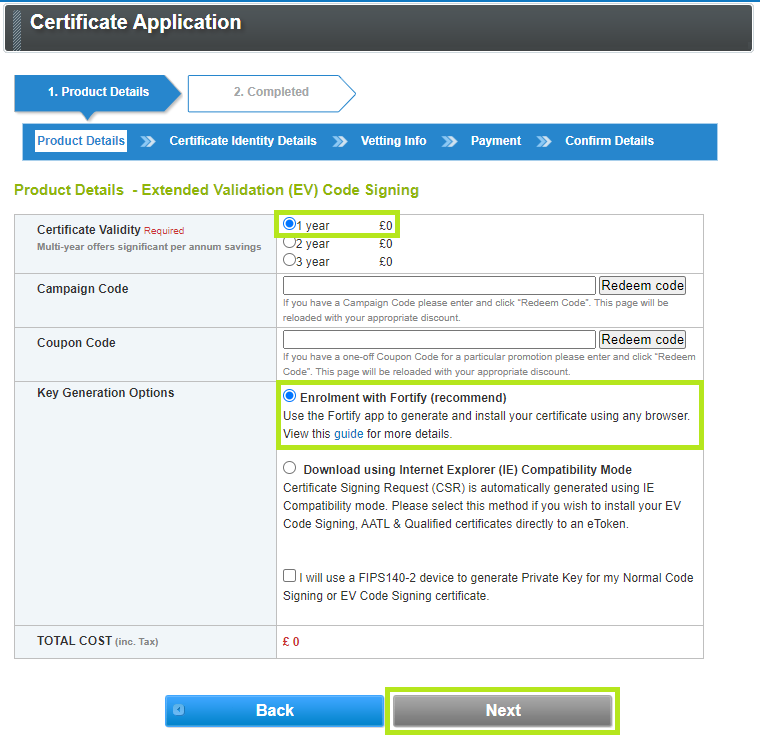This screenshot captures a webpage from an unknown website, specifically from the "Certificate Application" section. The interface is organized with a dark gray banner at the top stating "Certificate Application." Underneath this banner, there are two steps indicated: "1. Product Details" (highlighted with a blue arrow) and "2. Completed" (marked with a white arrow).

Following the navigation banner, a blue section titled "Product Details" breaks down further steps and details required for certification. These subsections include "Certificate Identity Details," "Vetting Info," "Payment," and "Confirmed Details." Within the "Product Details" subsection, there are several specific parts to fill out or choose from:

- **Certificate Type Selection:** 
  - "Extended Validation (EV) Code Signing."
- **Certificate Validity Options:**
  - "Multi-Year Offer Significant Per Annum Savings," with options for one year, two years, or three years, all listed at zero pounds. The one-year option is selected.
- **Campaign Code Input:**
  - A field to enter a campaign code along with instructions to click "Redeem Code" for discounts, causing the page to reload to reflect the discount.
- **Coupon Code Input:**
  - A provision to enter a one-time coupon code with similar instructions for redeeming and reloading the page.
- **Key Generation Options:**
  - "Enrollment with Fortify (Recommended)," which is selected. Users can utilize the Fortify app to generate and install certificates using any browser.
  - An alternative method: "Download using Internet Explorer (IE) Compatibility Mode," automatically generating a Certificate Signing Request (CSR). This method should be reselected if installing EV Code Signing, AATL, and Qualified Certificates directly to an eToken.
  - A checkbox is available to confirm the use of an FIPS 140-2 device for generating a private key for normal or EV Code Signing Certificates.

At the bottom of the page, the total cost, including tax, is noted as zero pounds. Navigation buttons include a blue "Back" button and a gray "Next" button outlined in green.